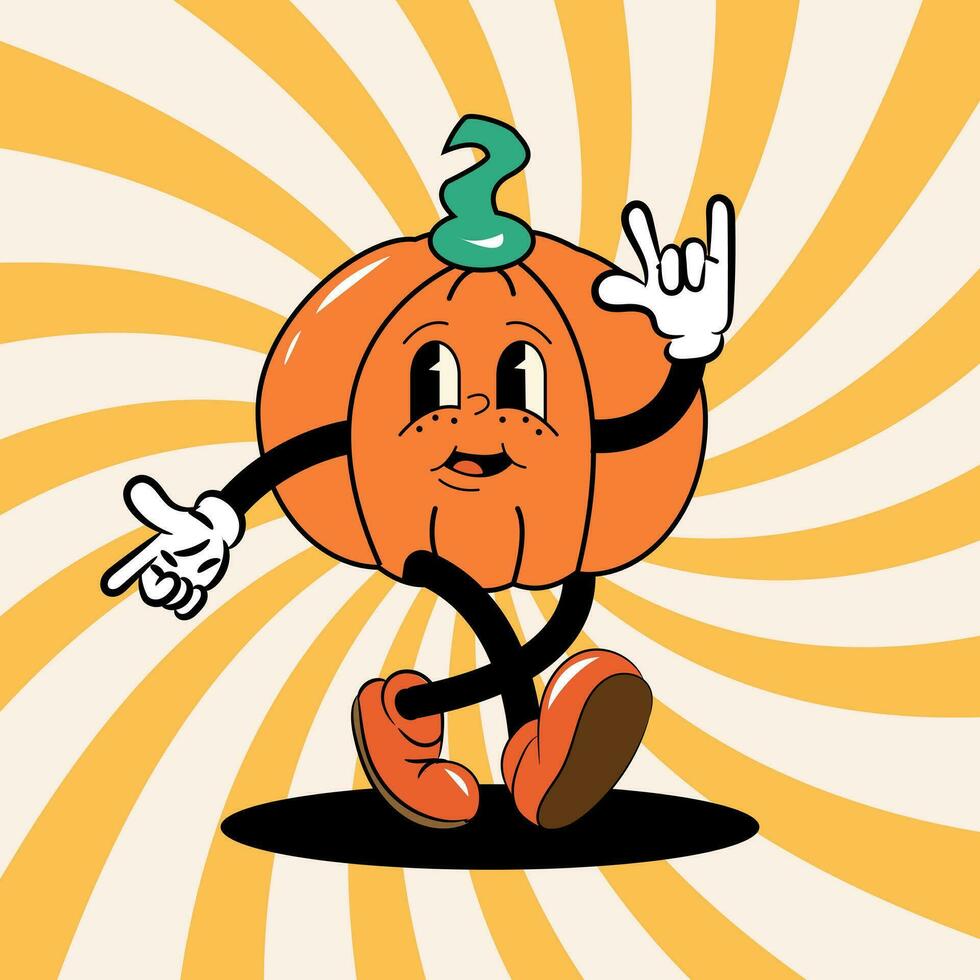This is a cartoon image set against a psychedelic, 1970s-inspired background, featuring spiraling patterns in light yellow, orange, and white that emanate from the center. The focal point is a lively pumpkin character with a green stem atop its head. The pumpkin is divided into three sections and has a classic cartoon shape, complete with large, expressive eyes that are half black, half white, a small nose, a cheerful, perky mouth, and six freckles.

The pumpkin boasts noodley, spaghetti-like arms and legs, each adorned with white gloves reminiscent of Mickey Mouse’s iconic hands. The left hand is held up, forming a peace sign, while the right hand points downward in a playful gesture. The pumpkin wears large, darker-orange boot-like shoes with brown soles.

Cast against the black oval that serves as its shadow or platform underneath, the pumpkin appears to be standing, adding a touch of old-time cartoon charm to its whimsical and animated demeanor.